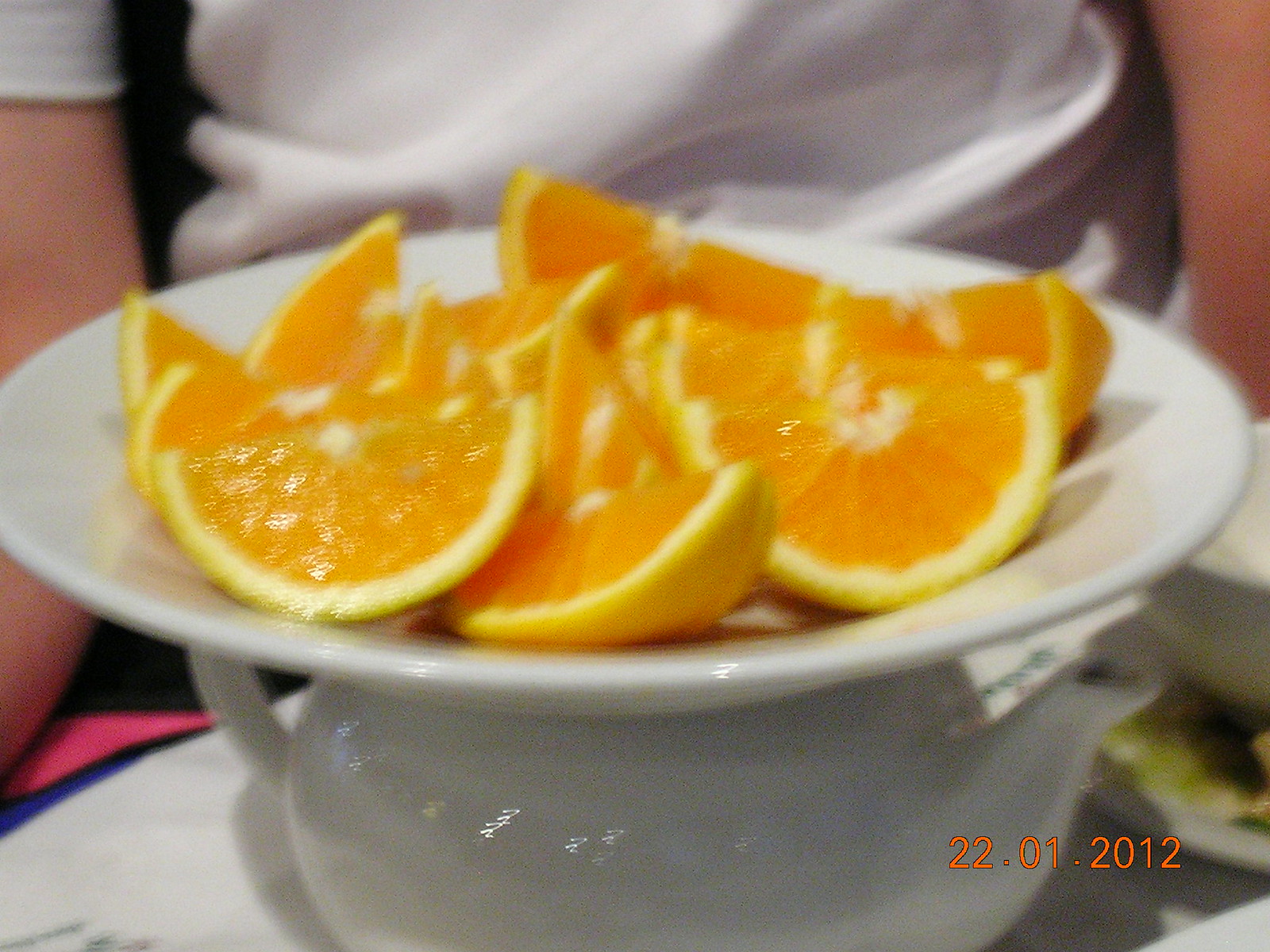A low-quality, blurry photograph captures a close-up of approximately 10-12 juicy, shiny orange slices arranged on a white plate. The plate is perched atop a white, porcelain teapot. Behind this setup, a figure with rumpled, white clothing is partially visible, including sections of their chest and bare arms to the right and left of the frame. It is indeterminate whether the figure is male or female. To the right of the teapot, another white bowl or plate can be seen, supported by what appears to be a patterned surface featuring multiple colors and possibly a white and hot pink design, though the details are unclear due to the blur. At the bottom right of the photo, the date "22.01.2012" is clearly displayed in orange numbers with a black outline.